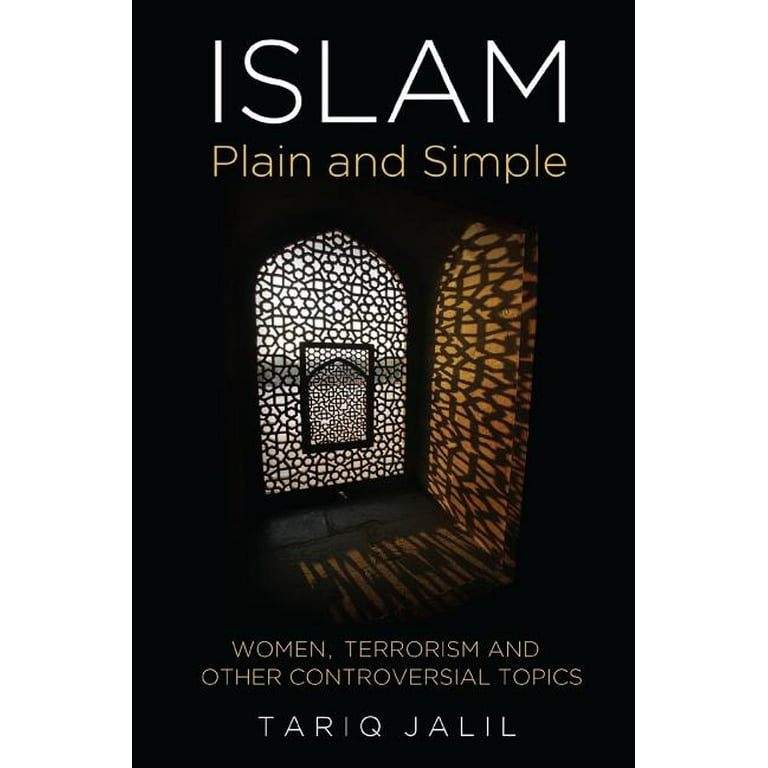The image is a book cover with a vertical rectangular layout and a black background. Dominating the center is a tall window with a distinctive shape — flat on the sides and bottom but arching to a point at the top. The window is adorned with intricately arranged black circles and includes a smaller vertical rectangle also filled with black circles. Goldish light filters through this window, casting intricate shadows on the brown wooden surfaces of the room inside. At the top of the cover, bold white text reads “ISLAM.” Below this, in a smaller, light yellow font, it says “Plain and Simple.” Further down, it lists the topics “Women, Terrorism, and Other Controversial Topics” in white, and finally, under this, centrally aligned, is the author's name, “Tariq Jalil,” also in white.